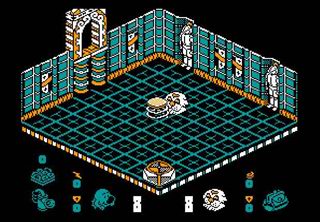The image showcases a detailed video game screenshot predominantly featuring a black background. Central to the image is a pixel-art style platform rendered in a 3D perspective, positioned at a 45-degree angle. This square platform appears wider than it is tall due to its orientation and features walls along the back, left, and right sides, forming an enclosed room. The walls, detailed with a blue coloration and white stripes, suggest an interior setting reminiscent of a castle. Intriguingly, these walls include inlets adorned with suits of knight's armor, depicted in white, and coat of arms that are black, white, and gold.

The floor of the platform is a black grid, accentuated with blue outlines, giving it a structured look. At the center of this platform lies an enigmatic circular object accompanied by a creature-like figure that resembles a ghost, complete with eyes and a mouth. 

Below the platform, various UI elements are displayed. Among these, a blue satchel icon outlined in black stands out alongside numerous other symbols. Interestingly, the same ghost-like creature from the platform reappears in these UI elements. Additionally, there are two eights spaced slightly apart, adding to the interface details. The combination of these elements paints a clear picture of a richly detailed and atmospheric video game setting.